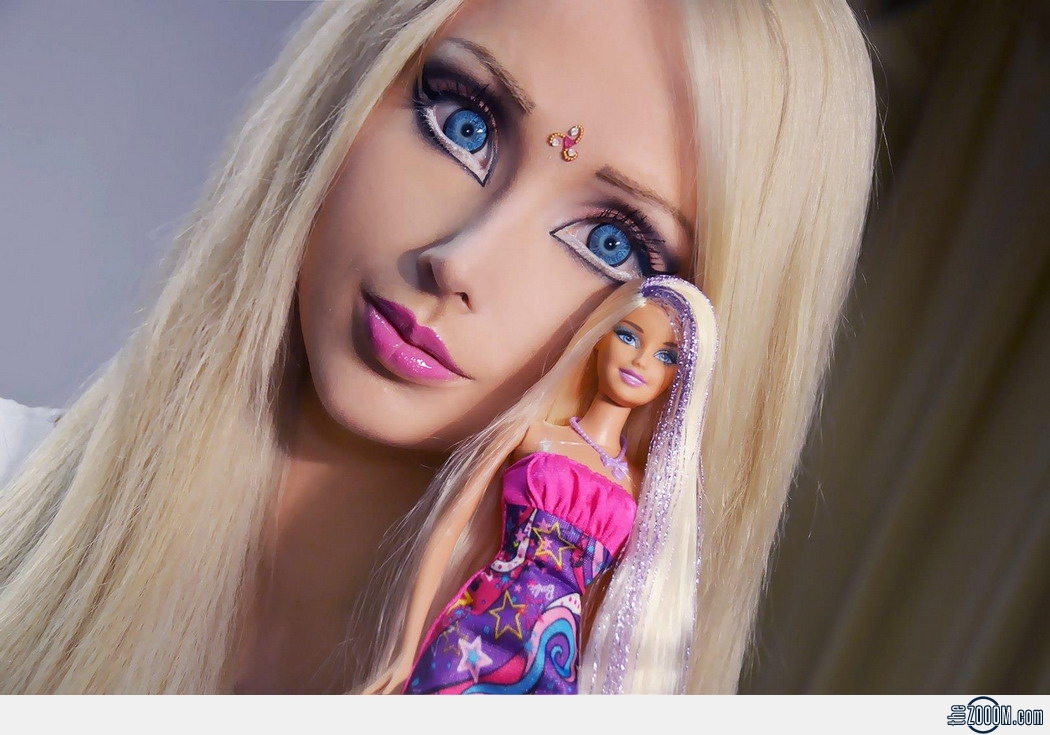The photograph showcases a woman with long, bleached blonde hair, styled with pink lipstick, pronounced eyeliner to make her eyes appear larger, and vibrant blue contacts. A small three-armed gem adorns the center of her eyebrows. Wearing a white top, she holds a Barbie doll that bears a striking resemblance to her with similar blonde hair and exaggerated features. The Barbie is dressed in a pink halter top with a colorful, cosmic purple design featuring stars, stripes, and swirls. The photograph is taken at an angle, cutting off part of the woman's head so that the top points towards the top-right corner. The image, possibly with an AI-generated effect, evokes an uncanny valley sensation due to the woman's doll-like appearance. A "zoom.com" watermark is visible at the bottom of the image.